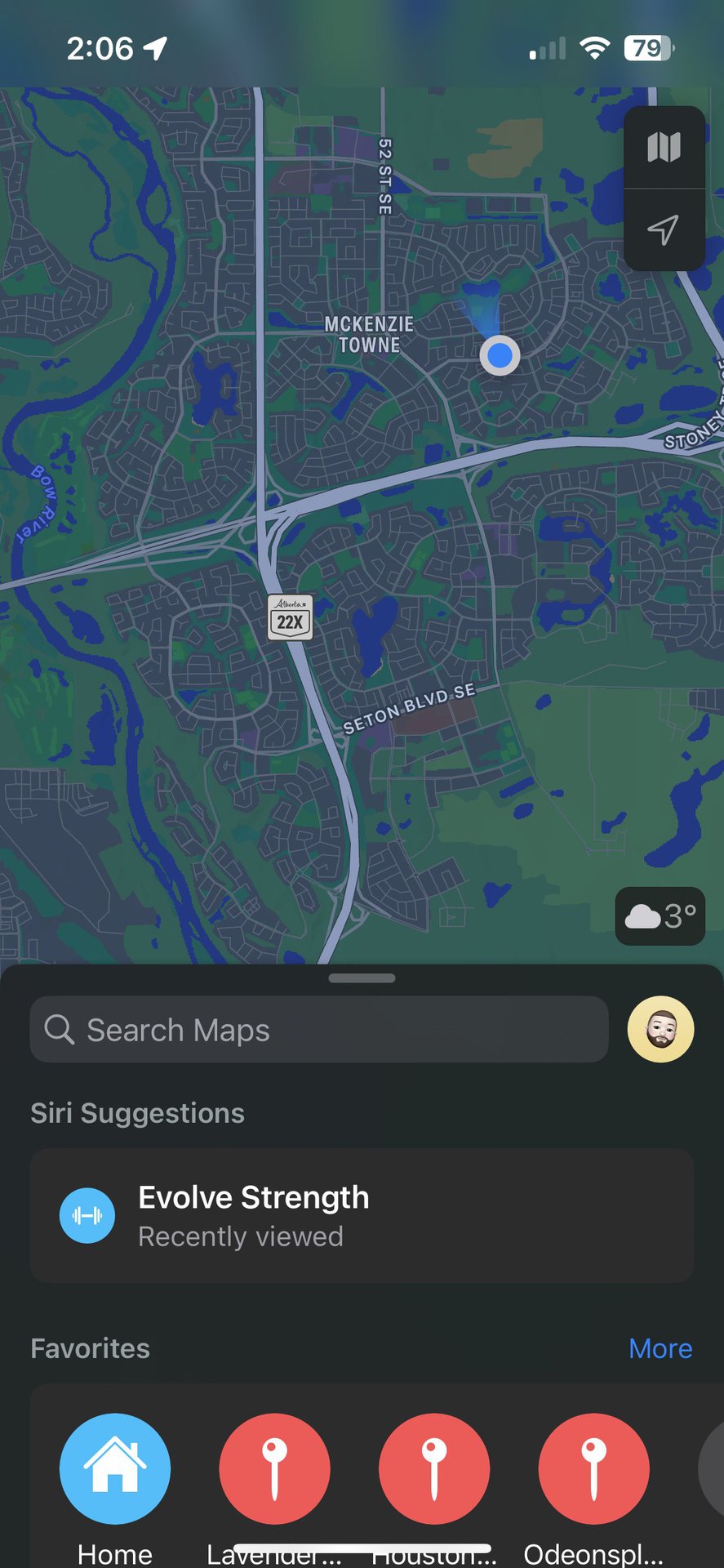This screenshot, captured on a mobile phone, displays a Google Maps interface focused on the area around Evolved Strength in McKenzie Town. At the top of the screen, the time is indicated as 2:06 PM, with standard icons for phone service, WiFi connectivity, and a 79% battery life. The map itself is rendered in shades of blue and green, showcasing the geographical layout and major routes, including Highway 22X that traverses the center of the map.

An indicator pinpoints the location of Evolved Strength along a prominent street in McKenzie Town. At the bottom of the map, there is a weather icon displaying a temperature of 3 degrees, suggesting the current local climate.

Beneath the map, a menu toolbar is visible with the option to "Search Maps." The section titled "Siri Suggestions" highlights that Evolved Strength was recently viewed. At the bottom of the image, a "Favorites" list is shown, featuring locations such as "Home" in blue, "Lavender," "Houston," and another personalized location marked in red.